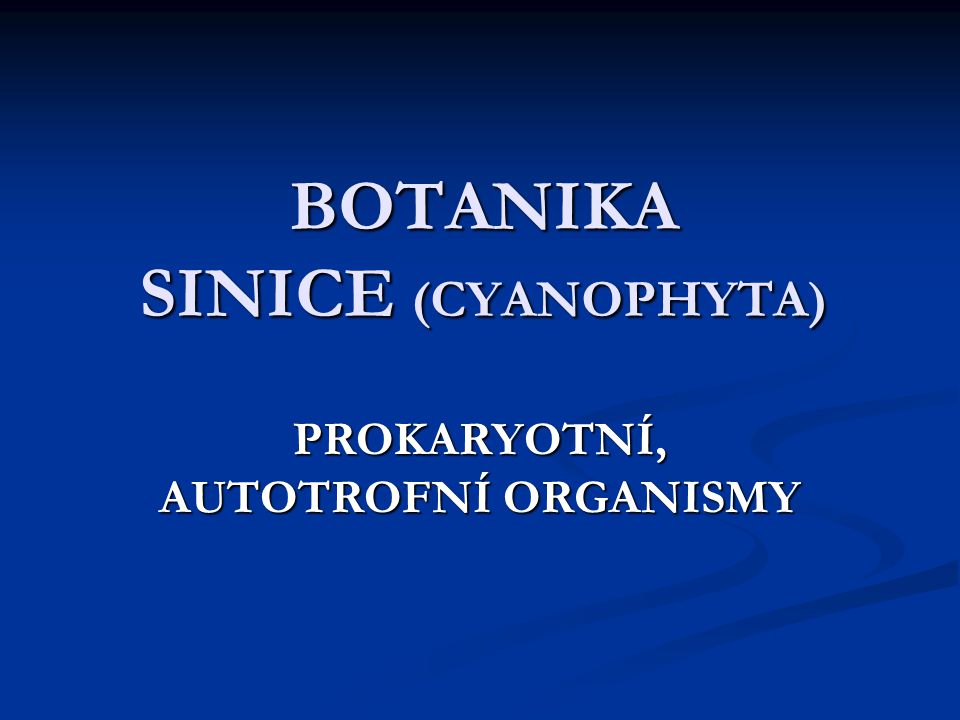The image is a landscape-oriented rectangular slide with a gradient background that transitions from dark blue at the top to a lighter blue towards the bottom. In the lower right, there are decorative darker blue swirls within the lighter blue area, adding a visual effect. Overlaying this background is white, all-caps serif font text with a black shadow for emphasis. 

The text, likely in an Eastern European language, is arranged in four lines. The first line reads "Botanica" followed by the second line "Sinice" (S-I-N-I-C-E), with "cyanophyta" written in parentheses. The third line, after a space, says "Prokaryotni" (P-R-O-K-A-R-Y-O-T-N-I) and the fourth line "Autotrofni Organismi" (A-U-T-O-T-R-O-F-N-I O-R-G-A-N-I-S-M-Y). The top three words before the parenthesis are slightly larger than the text below. This design and content suggest it may be part of an introductory slide for a biology presentation, focusing on cyanophytes, prokaryotes, and autotrophic organisms, potentially for a university-level course.